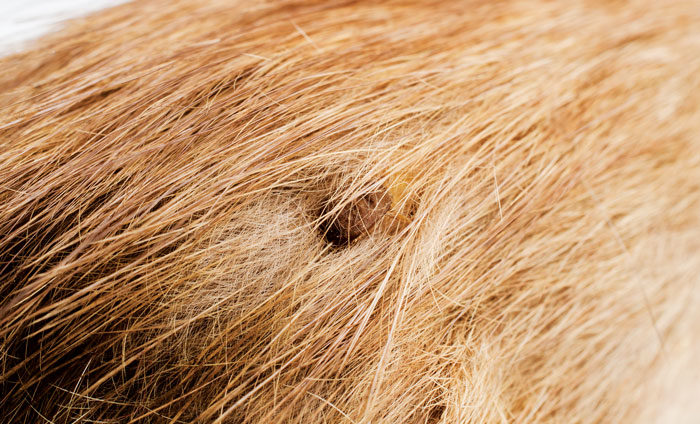This is a horizontally aligned rectangular close-up image of what appears to be medium to light brown animal hair, possibly from a dog. The entire picture is filled with this coarse and slightly wavy hair, with a notable blurriness along the right side. The hair color transitions to a darker brown shade in the lower left corner, possibly due to the camera angle. Toward the center of the image, there's a small, circular, darker brown knot or cluster of hair. This knot, which looks somewhat indented, stands out against the lighter surrounding hair. The background of the image has a white to light blue hue, contrasting the warm tones of the hair. This detailed focus on the hair suggests a natural, almost random element within the dense texture.